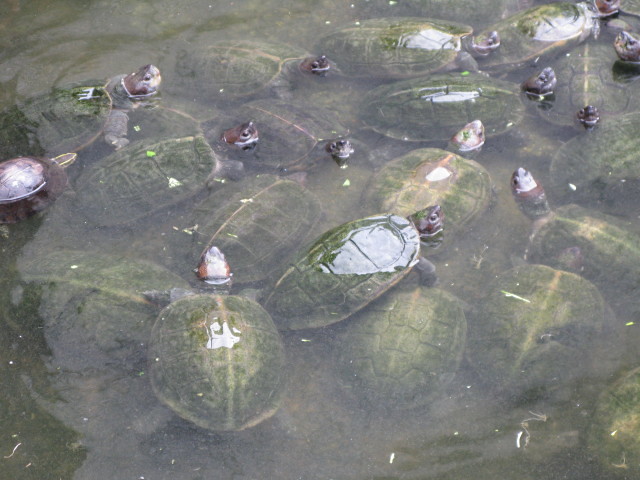The image captures a serene scene of numerous tortoises swimming in a shallow, slightly brown-tinted body of water. The water appears somewhat foggy, yet clear enough to reveal the green, yellow-striped shells of the tortoises below. Many tortoises are partially submerged, with their small, light and dark gray heads poking above the water, seemingly gazing upwards. The sunlight illuminates their shells, highlighting the intricate yellow lines and the lighter green hues in the center of their backs. Amidst what appears to be a group of around 30 tortoises, some are fully submerged yet still visible through the shallow water, adding to the peaceful ambiance of the scene.